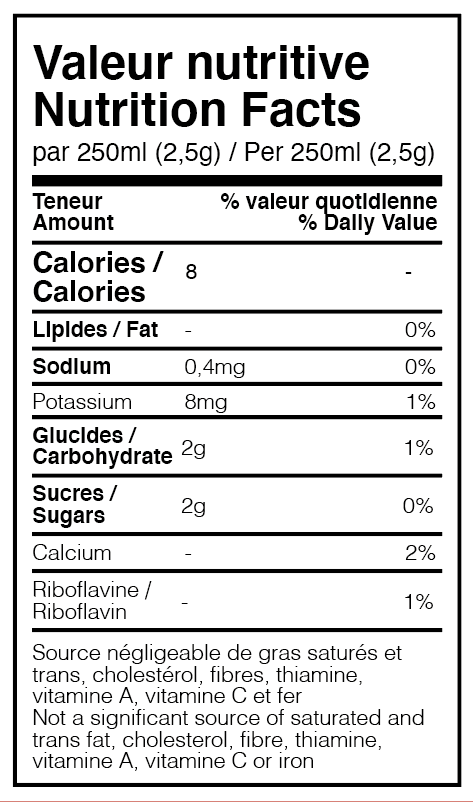This image displays a bilingual (French and English) nutritional facts label, set within a large white rectangular background bordered in black. At the top, it lists "Valeur nutritive" in French followed by "Nutrition Facts" in English. The values provided are for a 250 ml serving size, denoted as "par 250 ml" and "per 250 ml."

Key nutritional information is detailed in both languages, including:

- **Calories / Calories:** 8
- **Lipides / Fat:** 0% 
- **Sodium / Sodium:** 0.4 mg (0%)
- **Potassium / Potassium:** 8 mg (1%)
- **Glucides / Carbohydrate:** 2 g (1%)
- **Sucres / Sugars:** 2 g 
- **Calcium / Calcium:** 2%
- **Riboflavine / Riboflavin:** 1%

The label also notes that it is not a significant source of saturated and trans fats, cholesterol, fiber, thiamine, vitamin A, vitamin C, or iron.